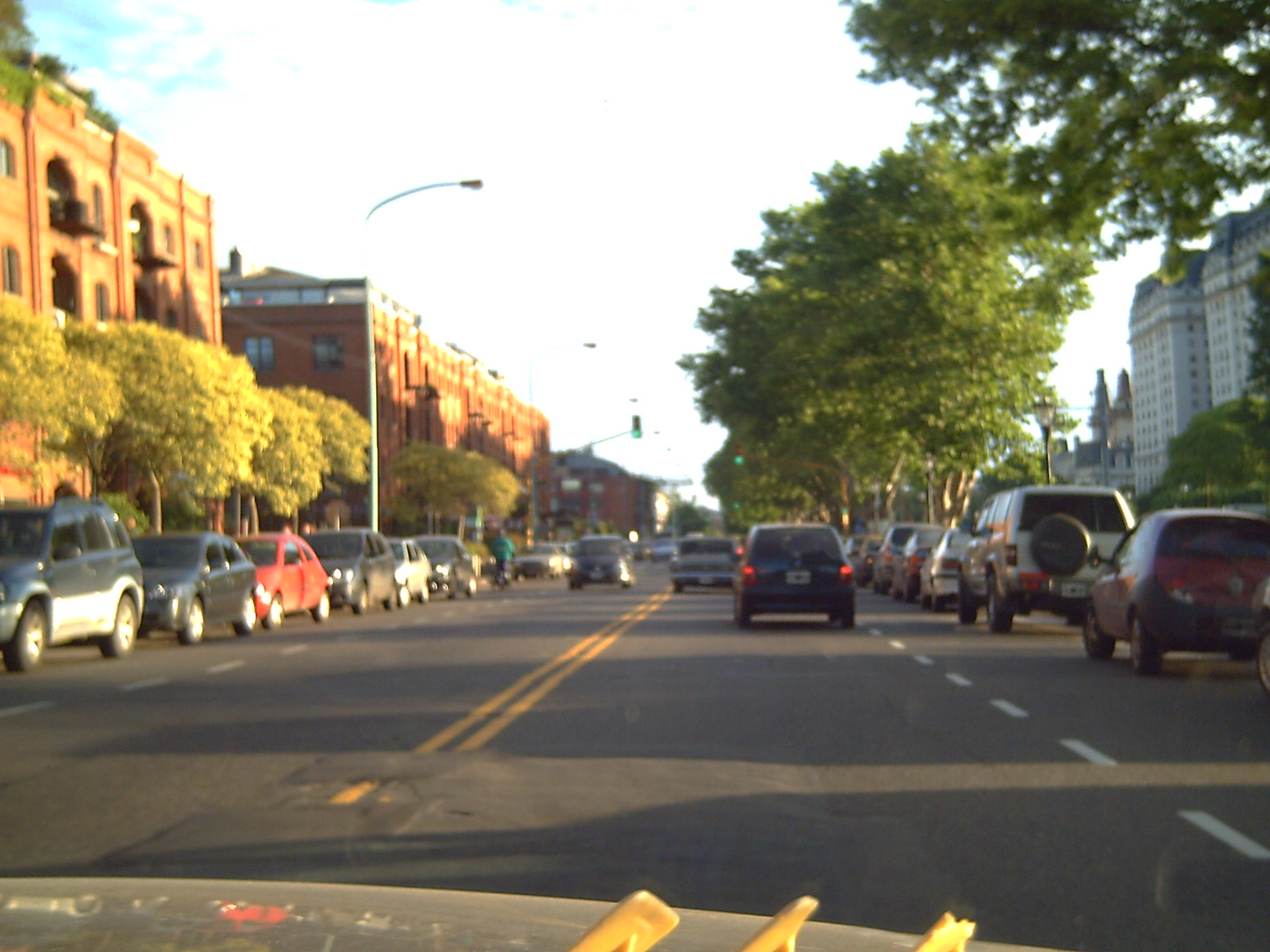The image captures a bustling downtown street from a first-person perspective, seemingly from someone sitting in the passenger seat of a car. The hood of the car is visible at the bottom, setting the scene from a low angle. The street is lined with several lanes of traffic, marked by a solid yellow line in the center and striped white lines on the sides. Cars are parked along both sides of the street, and directly in front of the viewer, there's a small blue car with its brake lights on. In the opposite lane, a dark car approaches from a distance. 

The urban landscape is rich with large multi-story buildings, including some red brick structures about three stories high and one with steep, tall edges that could be a church. Tall, leafy trees line both sides of the street, indicating it's summertime, their green canopies creating a lush corridor. Overhead, the sky is mostly blue with a few white clouds, suggesting a bright daytime setting. Hanging streetlights and a visible green traffic light in the distance add to the street's busy ambiance, while a person midway down the block appears to be getting into a car. This vibrant scene is characteristic of a lively downtown area, possibly near a college campus or apartment buildings.